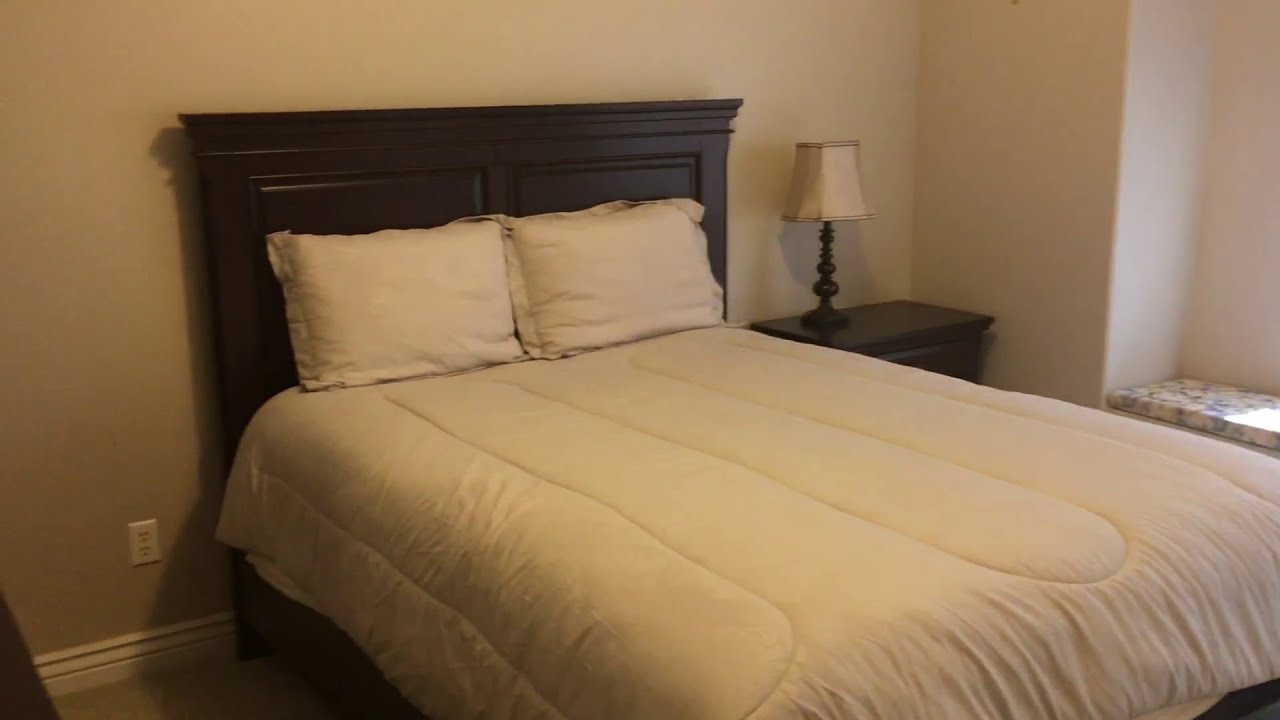This image resembles an advertisement for a hotel bedroom. Dominating the center is a large, neatly made bed, likely a queen size, draped with a light-colored comforter and accented by two oversized white pillows. The bed features a dark wooden headboard and is set against a background of cream-colored walls with white baseboards. To the right of the bed stands a wooden bedside table topped with a lamp, characterized by its candelabra-style base and white lampshade. The carpet beneath appears to be a light beige or gray, and to the right, there seems to be an alcove suggesting the presence of a window with a marble sill, though the actual window is not visible. The entire setting conveys a modest yet comfortable hotel room decor with hues of off-white, tan, brown, and a touch of dark brown, indicating a thoughtfully designed indoor space.